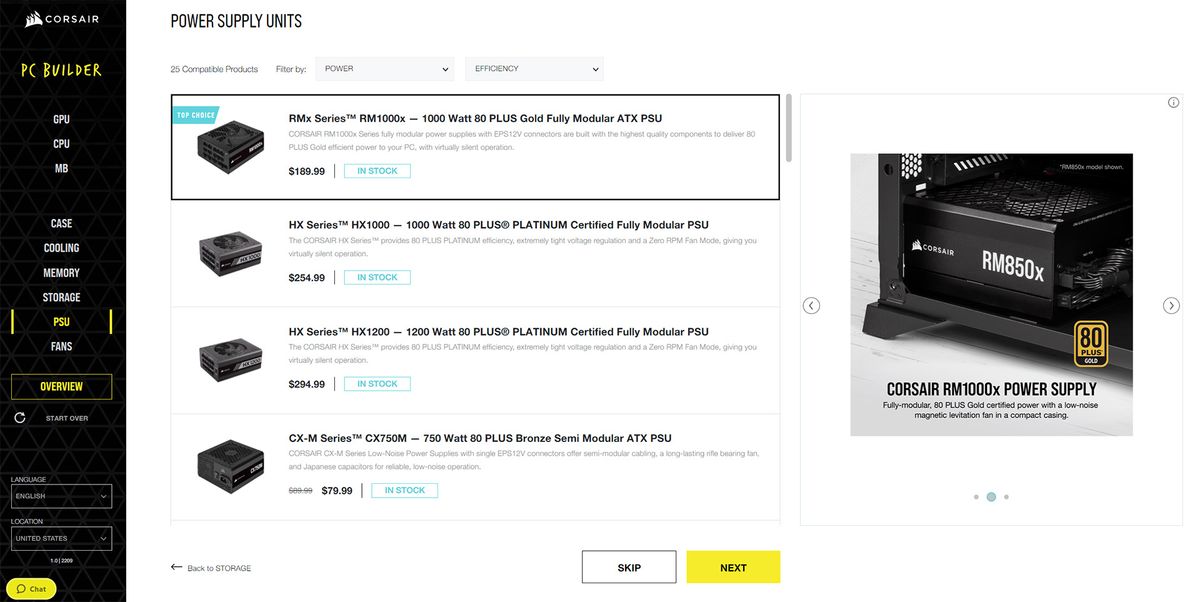This image is a cropped screenshot from the Corsair website, specifically highlighting its information about power supply units (PSUs). The layout features a black-background navigation menu on the left with white and yellow text. The currently selected menu item is PSU, which stands for Power Supply Unit, indicating that this is a section of the website dedicated to these components essential for building PCs. The site offers various PC components for purchase.

To the right of the navigation menu, there is a list of four different power supply units, each accompanied by a small thumbnail image, a title with a brief description, and the price. Below each product listing, there's an "in-stock" alert indicating availability. Dominating the far right-hand side of the screenshot is a larger, prominently displayed image of a Corsair RM1000X power supply unit, which is clearly being advertised. This emphasis suggests that the RM1000X is a featured product, likely promoted due to its specifications or popularity.